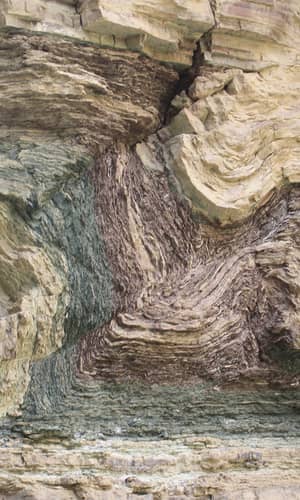The photograph captures a detailed close-up of an outdoor cliff face, showcasing a rich and textured expanse of layered rock formations. The intricate indentations and grooves are clearly visible, revealing the rugged texture of the rock. The composition is marked by distinct horizontal and vertical layers of varying colors, including sandy earthy tones, cream, and patches of grays. A prominent crack near the top adds to the dramatic geological features. Central to the image is an L-shaped seam of green that intersects the middle of the rock face. Above this green seam is a dark red band, followed by the typical sandy tones, and another reddish band on top, forming intricate L-U shapes. These formations highlight the natural geological processes that sculpted this landscape, giving it an almost abstract appearance, reminiscent of intricate patterns found in nature, such as the layered textures inside a brookie (brownie-cookie). The overall impression is that of a towering cliff edge, bathed in natural light, with an array of colors and patterns that tell the story of the earth's history.